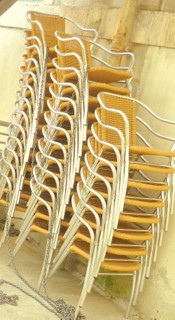The image shows three stacks of outdoor chairs, each with a white metal frame and light brown woven seats and backs. The stacks form a hierarchical arrangement, with the tallest at the back and the shortest closest to the camera, each stack holding approximately 10 chairs. The chairs are stacked neatly against a worn, dirty wall that features black marks and possibly mildew, suggesting an outdoor poolside or patio setting. The gray floor beneath them enhances the weathered appearance. Chains loosely wrap around the chairs, likely to prevent theft or to secure them when not in use. The overall shot appears slightly tilted, giving the stacks a forward-leaning look. The photo conveys a sense of the chairs being hastily arranged, perhaps moved out of the way for an event.